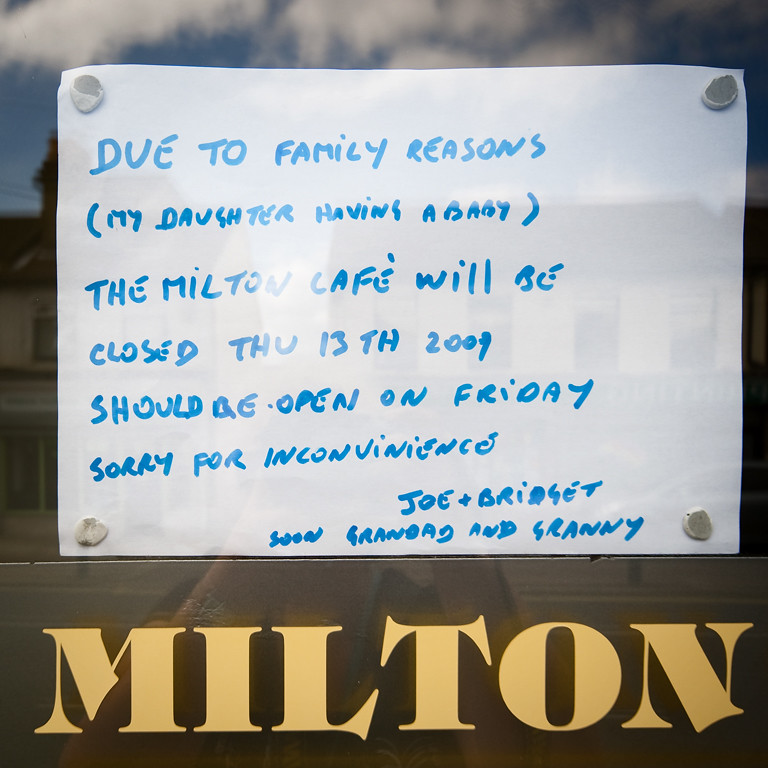In this photograph, a handwritten note is prominently displayed on the window of an establishment secured with wall putty at all four corners. The note, written in blue marker on a white piece of paper, reads: "Due to family reasons (my daughter having a baby), the Milton Cafe will be closed Thursday, 13th, 2009. Should be open on Friday. Sorry for the inconvenience. Joe and Bridget, soon Granddad and Granny." The note indicates that Joe and Bridget, the owners of the cafe, are temporarily closing the business to celebrate the birth of their grandchild. Reflected in the window are overhanging roofs and neighboring buildings, adding depth to the scene. Beneath the note, the name "Milton" is boldly displayed in large, yellow block letters, possibly as part of the store's signage.